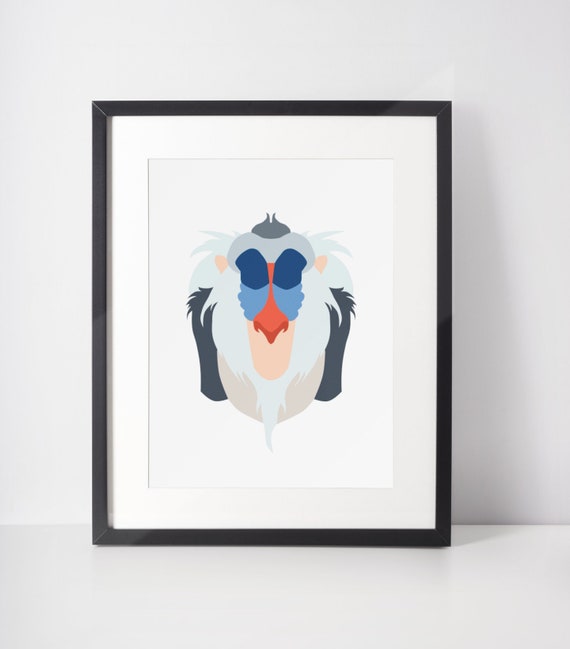This is a photo of a framed artwork featuring a character resembling a baboon from The Lion King. The frame is black and sits on a light white or light gray surface, leaning against a light gray wall. The artwork is accented by a white bevel mat and a light gray border that lines the right and bottom edges, extending halfway along the top. The centerpiece is a simple, two-dimensional painting with solid colors. The character has a round dark gray cap atop its light gray head, accented by a couple of hairs. It has big dark blue eye sockets with a thin red line down the center, forming an orange-red nose. Light blue shades appear under the eyes, while peach hues color the tiny ears and chin. The character's face also features white hair resembling sideburns, extending into a pointed beard. Gray shoulders, with hair sprouting from the top and sides, frame the lower part of the face.